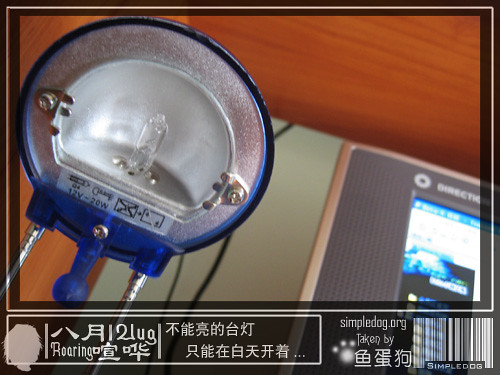The photo features a close-up view of the underside of a round lamp. The lamp has a silver metallic interior, bordered by a dark blue, plastic-like material. Inside the circular shade, which covers approximately three-quarters of the circle with a flattened bottom part, there's a tiny, inch-long light bulb that is currently off. This fixture is attached to two thin white poles coming from the bottom left corner, connected by a small bolt to the blue border.

Surrounding the lamp, the background reveals a wooden ceiling and a pale green wall. To the right side of the image, there's a partial view of a computer or TV screen, encased in a grayish frame, displaying an indistinguishable image. At the bottom, just below the lamp, there's a black bar intersected by a white rectangle filled with various Asian characters and a barcode, with additional smaller text observed. Simpledog.org is also faintly visible among the text.